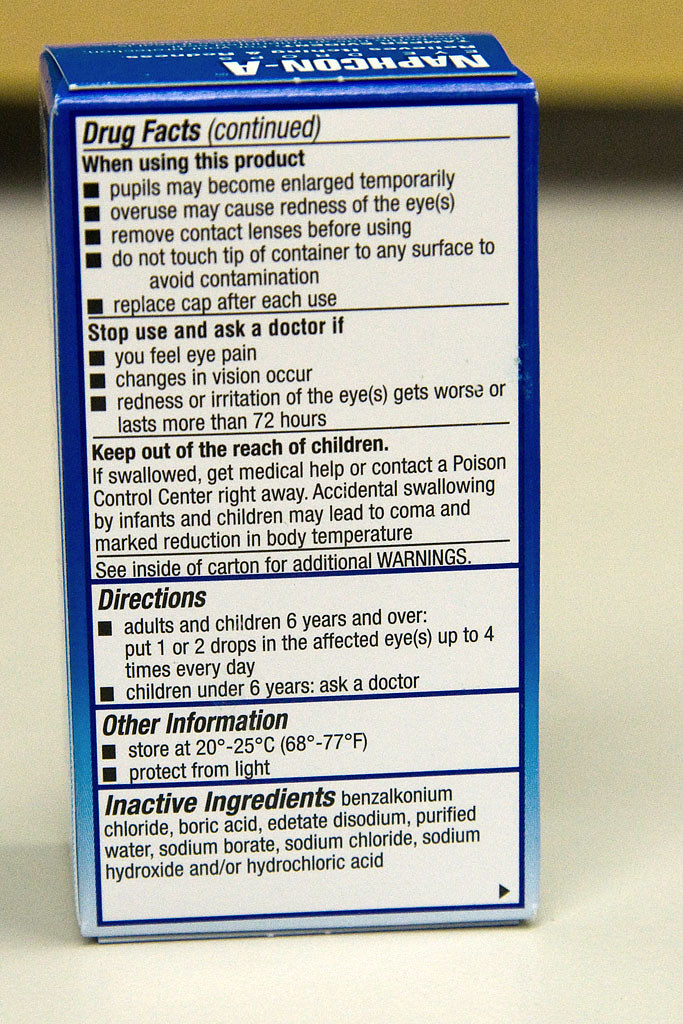The image is a close-up photograph of the back side of a rectangular, cardboard box for Nafcon A eye drops, set on a white countertop. The box features a color gradient that transitions from a darker blue top to a near-white bottom. Prominently displayed are the detailed "Drug Facts," which include various sections such as "When Using This Product," noting that pupils may temporarily become enlarged and overuse can cause redness, alongside warnings about removing contact lenses before use and preventing contamination by not touching the container tip to surfaces. Directions for use specify that adults and children aged six and older should apply one to two drops in the affected eyes, while children under six should consult a doctor. Additional warnings advise keeping the product out of children’s reach and provide instructions on what to do if swallowed. The box also lists inactive ingredients under "Other Information" and advises storing the product at a controlled temperature and protecting it from light. The box is standing upright, allowing all this information to be clearly visible.